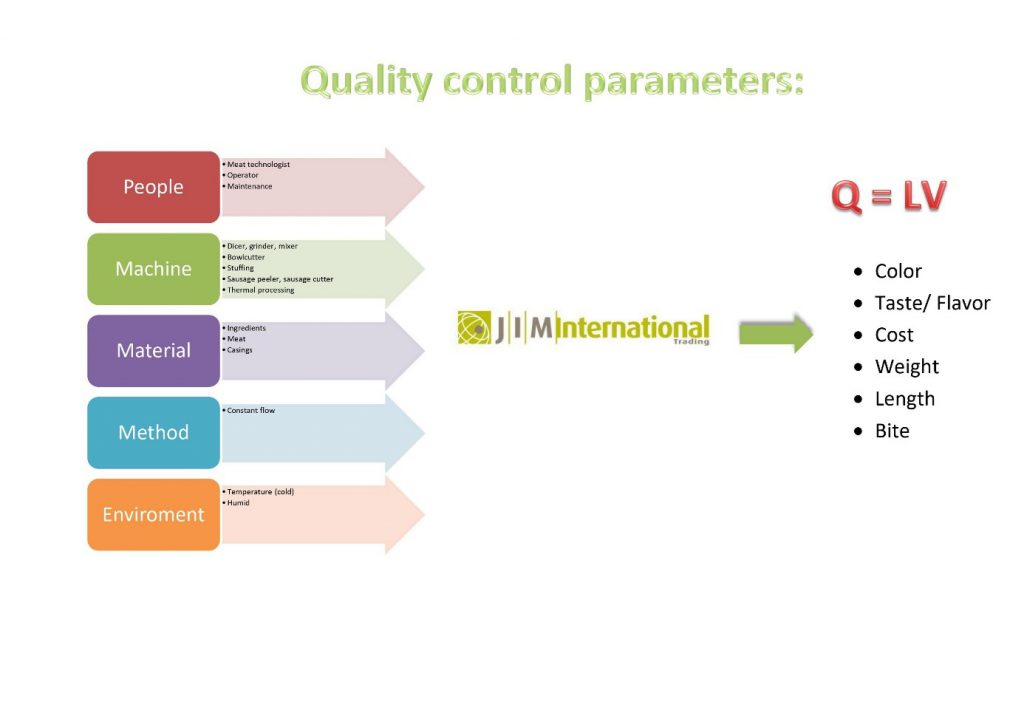The image features a detailed layout titled "Quality Control Parameters" at the top center in green letters, set against a white background. On the left side, there are five distinct categories represented by colored rectangles with curved edges: a red rectangle labeled "People," a green rectangle labeled "Machine," a purple rectangle labeled "Material," a pale blue rectangle labeled "Method," and an orange rectangle labeled "Environment." Each rectangle has a corresponding light-colored arrow pointing to the right, leading to a central logo that reads "JIM International Trading." Further details within these arrows are too small to be legible. From the central logo, an additional arrow points to the right side of the image, where the text "Q = LV" is prominently displayed in red. Below this, in black, is a list detailing essential quality control attributes: color, taste/flavor, cost, weight, length, and bite.